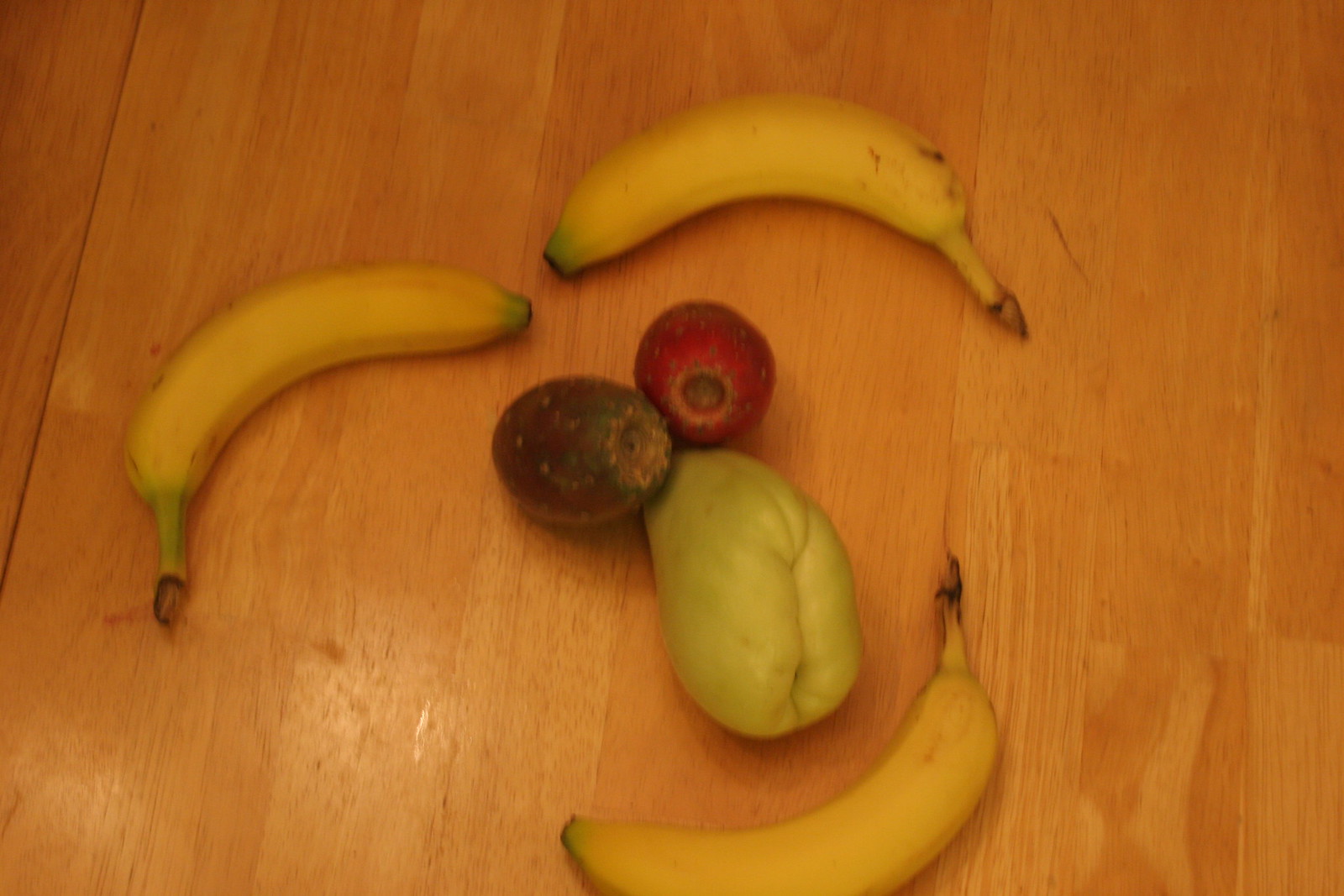On a light brown wooden table, a playful arrangement of fruits is designed to resemble a smiling face. Two ripe bananas, complete with stems — one yellow with a brown tip, one green with a brown tip, and a third yellow with a brown tip — are positioned lengthwise to form eyebrows. Below these, two spherical fruits, one purple and one green, are aligned side by side, mimicking eyes. These may be pomegranates, each featuring a distinct hole at one end. Centered beneath the 'eyes' is an oblong, unusually shaped tomato, simulating a nose. The bottom of the tomato is rolled inward, creating a prominent line that adds to its quirky appearance. Completing this whimsical face, a third banana, curved upward, imitates a broad, cheerful smile. Despite some bruising, the bananas' playful arrangement contributes to the overall endearing and creative look of the fruit face.